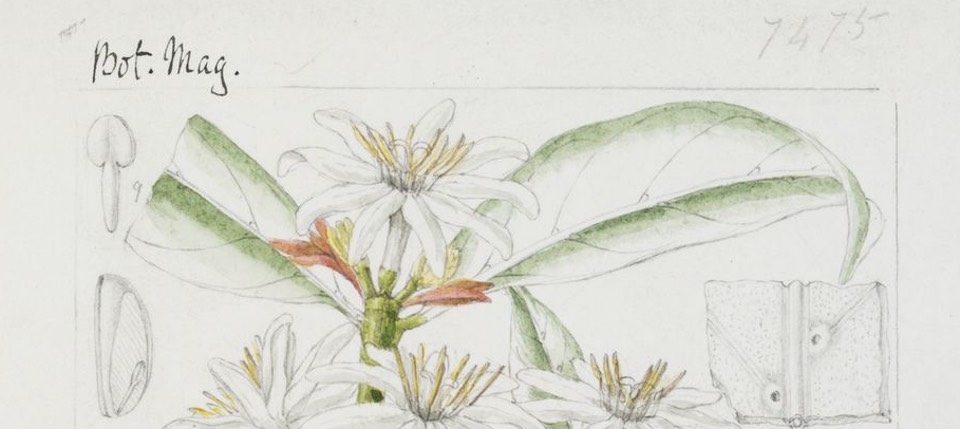The image showcases a meticulously detailed botanical drawing of a flower with part labels. The flower's background is stark white, emphasizing its vivid colors—green leaves, clusters of red petals at the bottom, and prominent white petals with tall yellow pistils and stamens at the center. The flower appears beautifully open and has an almost whimsical feel, with large leaves, particularly the one curling under on the right. On the drawing's right side, intricate gray pencil sketches illustrate various internal parts of the flower. Near the top right corner, the black text "BOTMAG" (B-O-T-M-A-G) and the number "7475" are visible. Below this, an image depicting seedlings emerging from the soil as roots grow upward is included. On the left side of the drawing, there is a small sketch of a shovel accompanied by the number "9," and on the right, an illustration resembling a book adds to the intricate details.